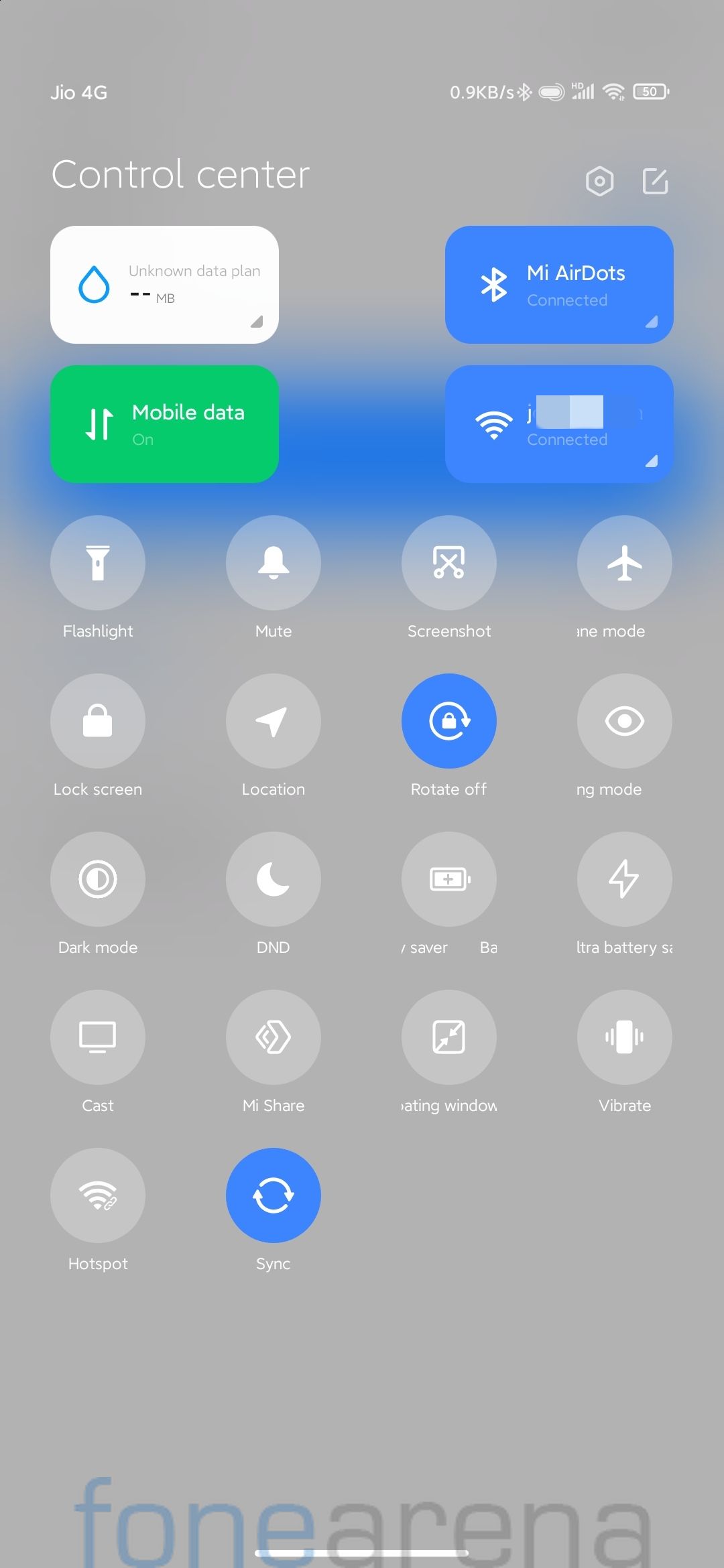This image is a screenshot captured from a smartphone, illustrating the device's control center and status bar. The background features a grey overlay, implying the presence of a secondary screen beneath the main interface.

At the top of the screen, the status bar exhibits various indicators: on the left, white text spells out "JIO" (capital "J", "I", "O") followed by "4G" (capital "G"). Moving rightward, it displays "0.9 KBS" (with "K" and "B" capitalized) alongside a forward slash and a lowercase "s". This is followed by icons indicating Bluetooth connectivity, a microphone, HD capabilities, signal strength, WiFi connection, and a battery symbol showing 50% charge.

Below, on the left, "Control Center" is written with a capital "C". Adjacent to it on the right, three icons are visible: a hexagon with a circle at its center, a square with a pencil in its center, and under the "Control Center", a white rectangle with softened corners that includes a teardrop-shaped or water drop icon. This icon indicates "Unknown Data Plan", specified as "blank blank MB."

Further down, there is an arrow icon indicating data upload and download activity labelled "Mobile Data On." Next is a blue icon for Bluetooth connectivity displaying "My Air Dots Connected," followed by a WiFi icon with the label "Connected," accompanied by blue tabs.

The control panel then features various functional icons: 

1. Flashlight 
2. Mute 
3. Screenshot 
4. Airplane Mode 
5. Unlock Screen 
6. Location 
7. Rotate Off 
8. Dark Mode 
9. Do Not Disturb (DND)
10. Battery Saver 
11. Cast 
12. My Share 
13. Rotating Window 
14. Vibrate 
15. Hotspot 
16. Sync